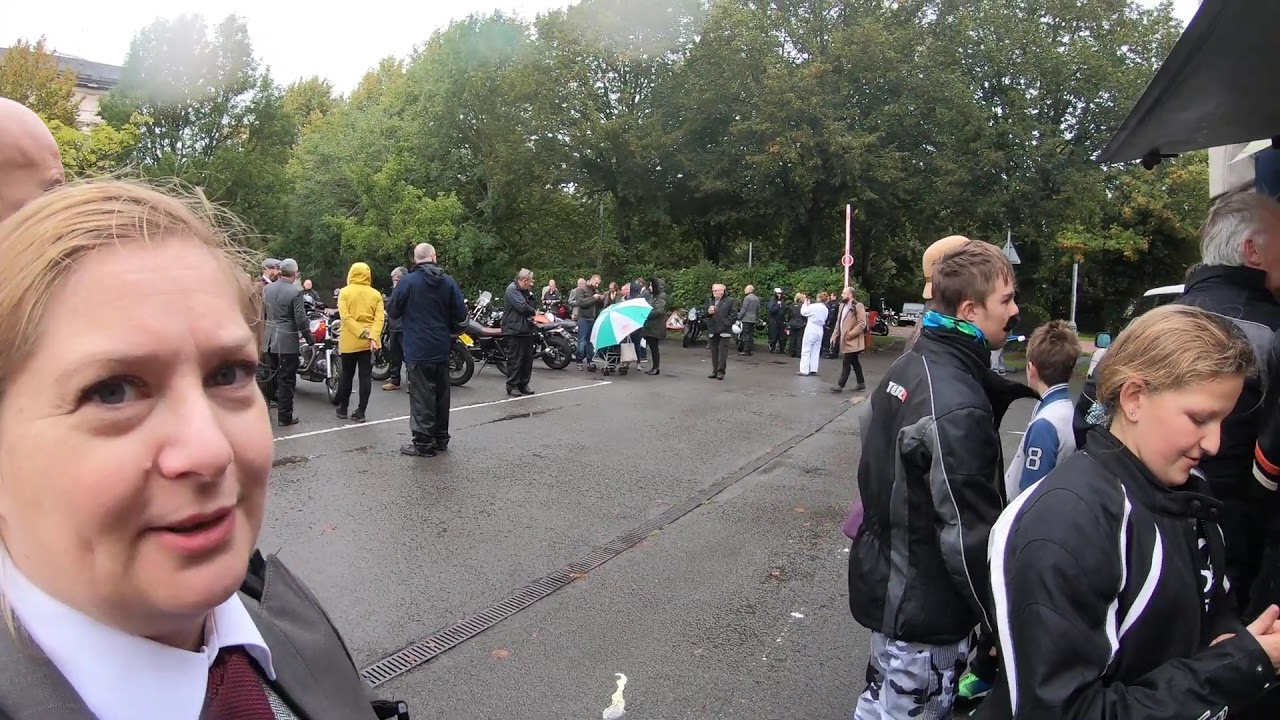This outdoor photo captures a rainy day scene with a wet road and an overcast sky. Prominently in the lower left is a woman with blonde hair pulled back, wearing a white collared shirt and red tie, looking directly at the camera. The setting appears to be a parking lot surrounded by tall trees and shrubs. A diverse crowd of people, including men, women, and children, are gathered, many donning black leather jackets. Among them, a child stands out in a blue and gray jacket with the number eight on the sleeve. Several motorcycles are lined up in the background. One woman in a gray jacket and an official in a green and white striped umbrella add to the scene evoking a sense of an organized event or parade. The asphalt path and nearby sidewalk indicate a structured outdoor space amidst the gathering crowd.